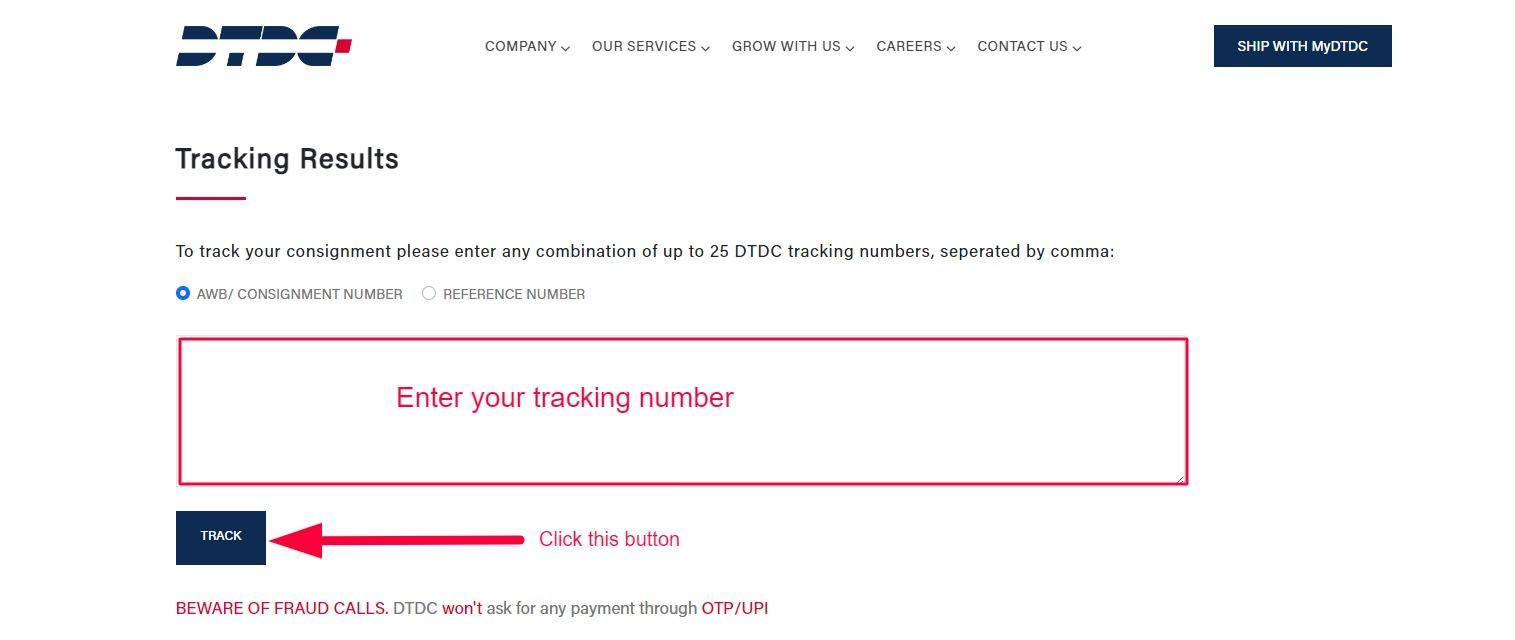In the image, the overall background is white, and the top section of the image features a blue header. On the top left corner, the icon "DTC" is displayed in dark blue. To the right of the icon, there are several navigation tabs labeled "Company," "Our Services," "Grow with Us," "Careers," and "Contact Us," each containing drop-down menus. On the top right part of the header, "Ship with My DTDC" is written in white text against the blue background.

Below the header, and beneath the DTDC icon, the words "Tracking Result" are prominently underlined in red on the left side. Directly below this, there are instructions saying, "To track your consignment, please enter any combination of up to 25 DTDC tracking numbers, separated by a comma."

Further down, on the left side of the image, there are two options for input: "AWB or Consignment Number" and "Reference Number," with the first option highlighted in blue. A pink-outlined space below this prompt instructs users to "Enter tracking number," with the text itself also in pink.

At the bottom left of the tracking input section, there is a blue "Track" button. A red arrow, pointing towards this button from the right side, has accompanying text that reads "Click this button" in pink.

On the lower part of the image, there is a cautionary message in pink and grey text which reads: "Beware of fraud calls. DTDC won't ask for any payment through OTP or UPI."